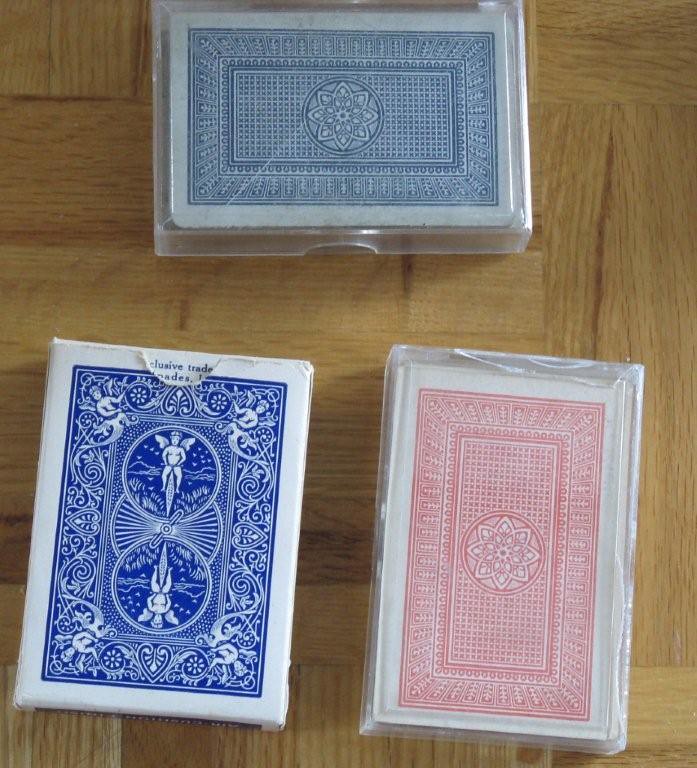In this detailed photograph, three distinct decks of playing cards are displayed on a wooden countertop composed of neatly arranged wooden planks. At the top of the image lies a deck encased in a clear plastic box, positioned horizontally. This particular deck features an intricate blue and white design on the back, characterized by a central mandala-like circle, surrounded by a detailed rectangle, which is further adorned by additional decorative elements.

In the lower right corner, another deck similar in design is visible, but with the primary colors switched to red and white, producing a striking contrast with the aforementioned deck.

Lastly, the lower left corner showcases a deck with a completely different design. This blue and white deck displays an ornate pattern featuring six angels or cupids. The central motif includes two vertically aligned circles, around which an elaborate scrolling design weaves, enhancing the overall aesthetic with its intricate craftsmanship.